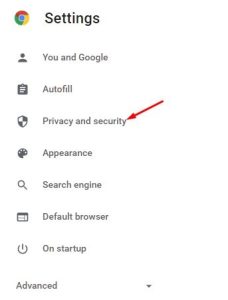A detailed description of the image could be:

This image appears to be a screenshot taken from a mobile phone, cropped to exclude the borders of the device, showcasing a white background with a neatly aligned series of menu options on the left. At the very top, a small Google Chrome icon is displayed, followed by the bolded black word "Settings." Below this, there is an expanse of white space leading to a gray person icon, symbolizing a user. Adjacent to this icon, the text "You and Google" is displayed. 

Further down, the word "Autofill" is listed next to an icon resembling a clipboard with lines, likely representing form fields. Directly beneath is a black and white shield icon, with the label "Privacy and Security," highlighted by a red arrow pointing directly at the 'Y' in "Security."

Following this, the word "Appearance" is visible next to an icon resembling an easel or painter's palette, symbolizing customization. Underneath, "Search Engine" is paired with a magnifying glass icon, indicative of search functions. 

Subsequently, the term "Default browser" is marked, aligned with an icon representative of this feature. Below this, "On startup" is noted alongside an on/off toggle switch, and finally, at the bottom, the word "Advanced" is accompanied by a drop-down arrow, indicating further options can be revealed.